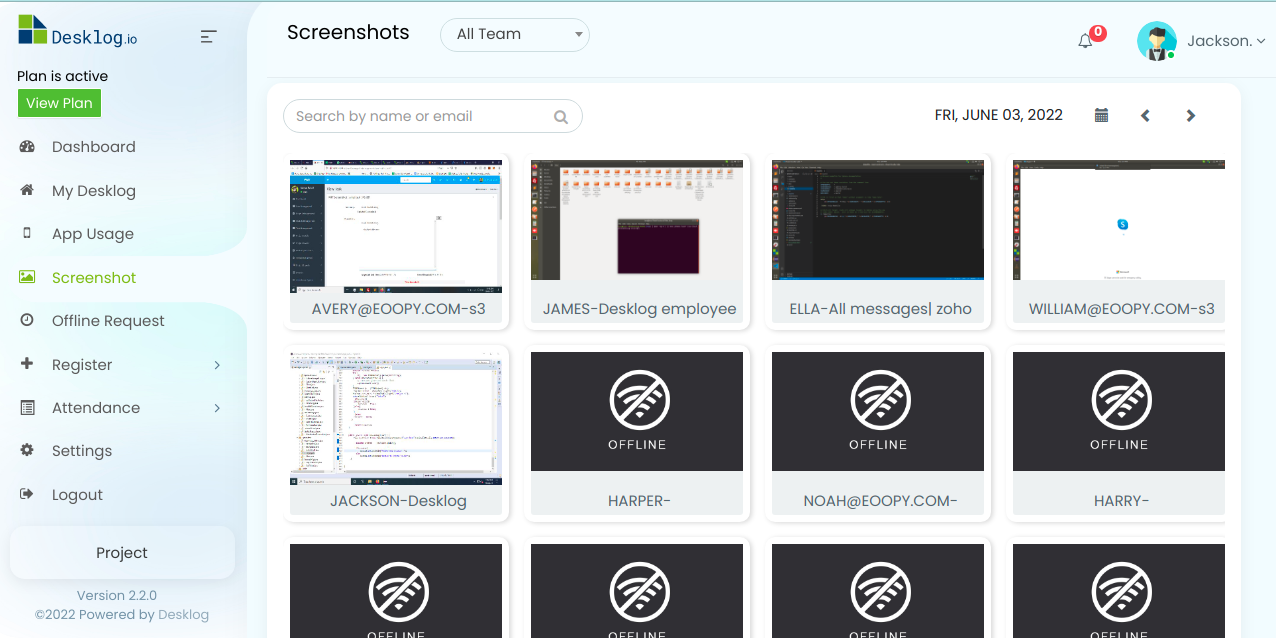The image is a screenshot taken from the website desklog.io, displaying a web interface for a productivity tool. At the top of the screen, there is a prominent label indicating that the plan is active, accompanied by a "View Plan" button in a green box. The left sidebar features an array of navigation icons paired with descriptions, listing options such as Dashboard, My Desklog, App Usage, Screenshot, Offline Request, Register, Attendance, Settings, Logout, and Project. At the very bottom of this sidebar, it is noted that the software version is 2.2.0, with a copyright notice for 2022 and a mention that the platform is powered by Desklog.

The main section of the interface focuses on screenshots associated with various team members. There is a search bar allowing users to search by name or email. The top of this section shows the word "Screenshots" with a filter option labeled "All Team." In the upper right corner, there is an icon of a cartoon person with black hair, attired in a vest and bow tie, labeled "Jackson." Next to this avatar is a notification area displaying a "0" within a red circle, indicating no new notifications.

Below, the screenshot thumbnails of different team members are listed. The names visible include Avery One, James (annotated with "desk log employee"), Ella, all messages Zoho, William E, WilliamEOB.com, Jackson (with the same avatar as mentioned earlier), Harper, Noah, and Harry. The lower part of the list is cut off, suggesting more entries below the visible screen area.